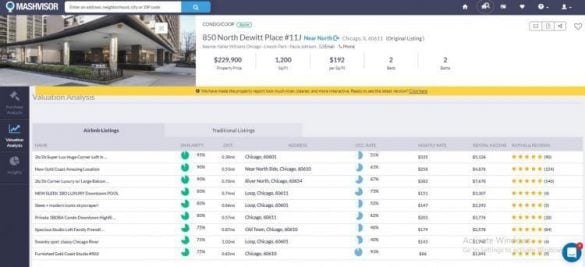Caption:

The website features a blue background with an indistinct name, possibly "Mash Manager." A search bar is prominently displayed, flanked by various small icons to the right, including one for settings. Below the title, there is an image of a modest office building with classical pillars and a covered entrance, surrounded by taller structures. The listing details include:

- Address: 850 North DeWitt Place, Unit LJ
- Price: $229,000
- Area: Approximately 2200 square feet

The text on the site is quite blurry, making it difficult to read most details. The page showcases a total of nine property listings, likely catering to those seeking to rent or purchase office space.